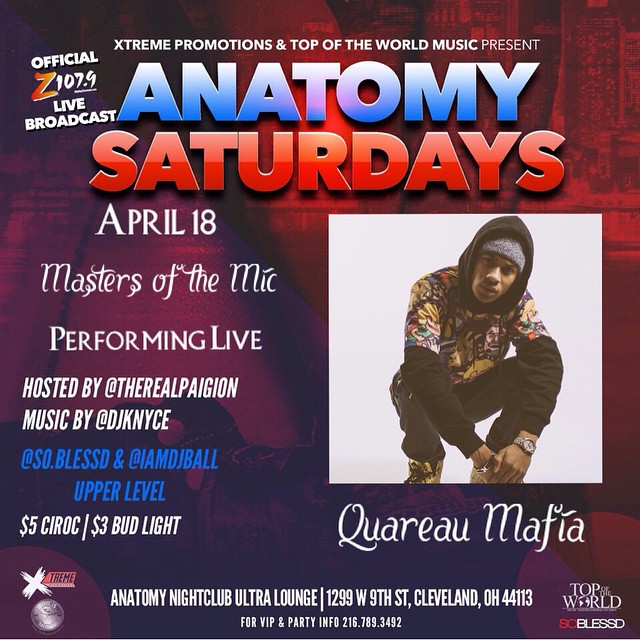This is a detailed flyer for the "Autonomy Saturdays" event at the Autonomy Nightclub Ultra Lounge on April 18th, located at 1299 West 9th Street, Cleveland, Ohio, 44113. The event is presented by Extreme Promotions and Top of the World Music, featuring an official D-107.9 Live Broadcast. The headline acts, titled "Masters of the Mic," will be performing live. The event is hosted by TheRealPirateGone, with music provided by DJ Canuts and I Am DJ Ball. The flyer prominently displays a photograph of a musician dressed in a hoodie, work boots, black pants, and a multicolored t-shirt, who will be performing live. Additional details include special promotions such as $5 Shorrock and $3 Bud Light. The poster's design features "Autonomy" in blue text and "Saturdays" in red text over a red-hued background. For VIP and additional party information, attendees are directed to call 216-789-3492 and TheRealPirateGone.